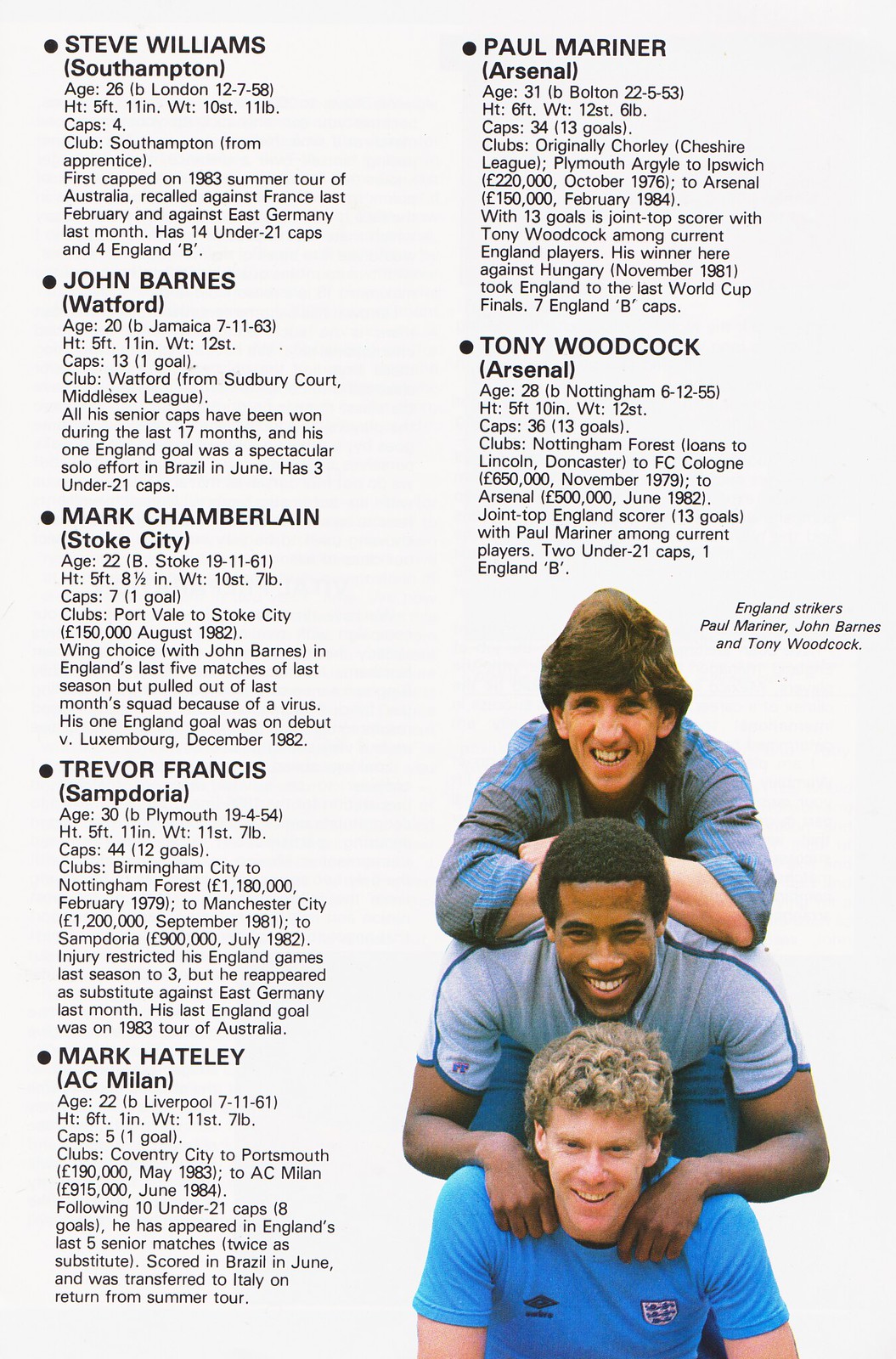The image is a detailed photograph of an article or program from a soccer match, featuring statistical information about several football players, including their names, clubs, ages, heights, weights, and first match details. Prominently displayed are the names: Steve Williams (Southampton), John Barnes (Watford), Mark Chamberlain (Stoke City), Trevor Francis (Sampdoria), Mark Hateley (AC Milan), Paul Mariner (Arsenal), and Tony Woodcock (Arsenal). 

In the bottom right corner of the page, there is a photograph showing three players posing together, all wearing blue shirts. The first player, with blonde curly hair and smiling, is kneeling at the front. Behind him, squatting slightly higher, is the second player with both hands fisted and resting on the first player's shoulders. The third player stands behind the second, leaning forward with his hands folded over each other and his elbows resting on the second player's shoulder blades. This trio consists of Paul Mariner, John Barnes, and Tony Woodcock, all of whom are England strikers. Their names are mentioned near the photograph, aligning with the detailed stats provided on the left-hand side of the page.